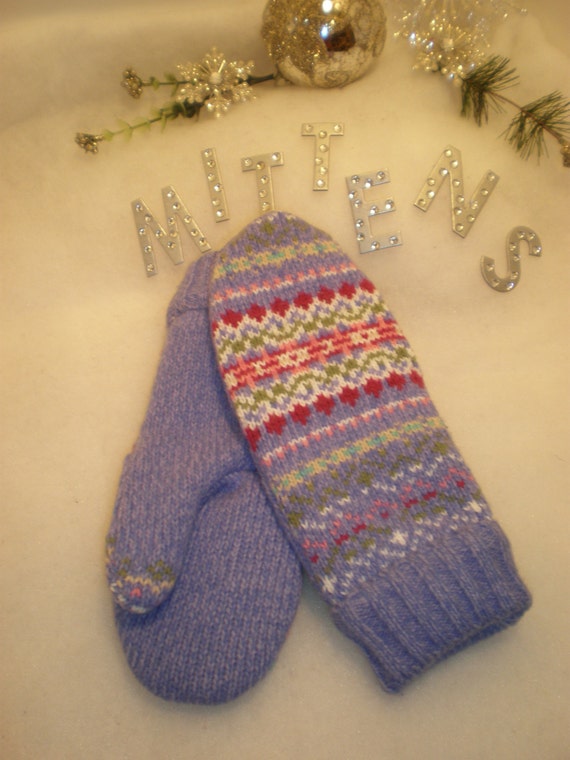The image is a winter holiday-themed photograph featuring a pair of hand-knit, feminine-looking purple mittens laid out on a white, cottony surface. The mittens are decorated with intricate patterns: the top side has alternating lines of yellow, pink, red, and green, possibly representing flowers with stems, while the underside is mostly purple with thumb areas adorned in yellow, green, and pink lines. Positioned centrally but slightly towards the bottom, the mittens draw your eye immediately. Above the mittens, the word "mittens" is spelled out in silver, bedazzled letters adorned with tiny plastic gems. At the very top of the image is a festive silver round Christmas ornament embellished with a glittery snowflake design. Flanking the ornament on the left is a green stem with gold plastic flowers, while on the right, a twig from a pine tree evokes the winter season. The overall color palette includes shades of pink, purple, red, light blue, white, black, gold, and green, enhancing the image's festive atmosphere. The setting and decorations clearly suggest it is taken during the winter holidays.